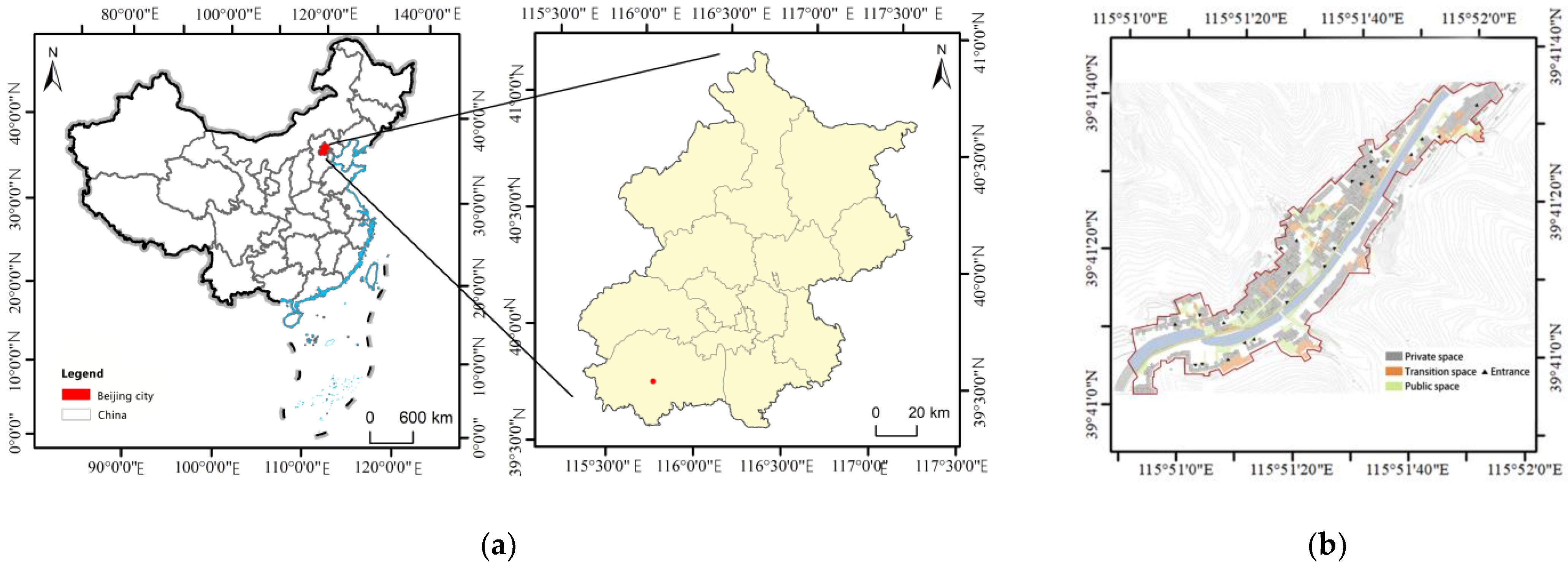The image displays a series of three digitally created maps arranged side-by-side, each within uniformly sized squares. On the left, there is a detailed map of China with all the provinces outlined, featuring a color-coded legend in the bottom left corner indicating 'Beijing City' in red and the rest of 'China' in white. The middle map zooms in to Beijing City, further dividing it into smaller regions or counties delineated by borders, against a consistent white background. Numbers marking the boundaries are present on all four sides. The rightmost map illustrates a long, possibly river-bound section within Beijing, segmented into various zones based on usage. The accompanying legend, placed in the bottom right corner, defines 'Private Space' in gray, 'Transition Space' in orange, and 'Public Space' in yellow. This array collectively outlines detailed geographical and functional divisions within China and Beijing through distinct color schemes, borders, and legends.